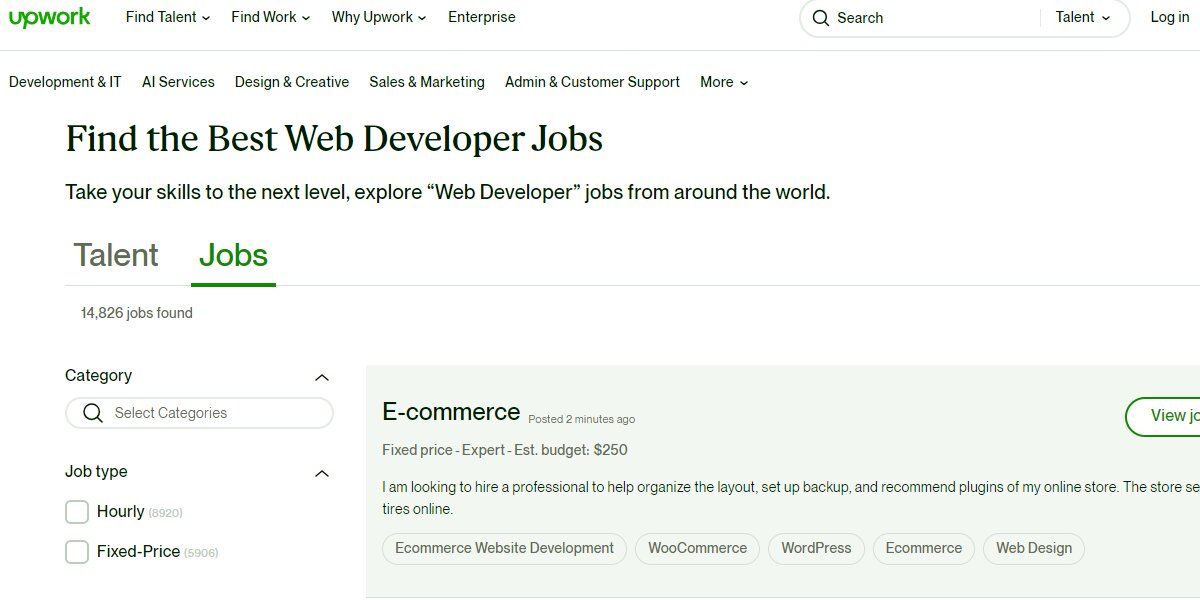**Detailed Caption:**

This image depicts a detailed desktop screenshot of the Upwork website, specifically showcasing its interface for job seekers and employers. The Upwork logo, represented in green, is prominently displayed at the top left corner of the page. A horizontal navigation bar stretches across the top, offering various options including "Find Talent," "Find Work," "Why Upwork," and "Enterprise."

Beneath the navigation bar is a search bar alongside a talent dropdown menu and additional dropdowns for "Find Talent," "Find Work," and "Why Upwork." Scrolling further down, several broad categories are listed, such as Development & IT, AI Services, Design & Creative, Sales & Marketing, Admin & Customer Support, among others.

The section presently displayed is focused on job opportunities for web developers, with a headline stating "Find the Best Web Developer Jobs. Take your skills to the next level. Explore web developer jobs from around the world." Users can toggle between viewing talent or job postings, with the current setting displaying "14,826 jobs found."

Further down the page, filtering options are visible: "Category," allowing users to select specific categories via search, and "Job Type," offering choices between hourly (8,920 listings) and fixed price (5,906 listings). A partial job listing is visible to the right, indicating an e-commerce opportunity posted just two minutes prior. The listing title includes "E-commerce," with a fixed price and expertise level required, indicating an established budget of $250. The job synopsis mentions seeking a professional to help organize the layout, set up backups, and recommend plugins for an online store, specifying skills in e-commerce website development, WooCommerce, WordPress, and web design.

This desktop view of the Upwork website offers a comprehensive look at how users can navigate to find or post jobs, emphasizing the functionalities and options available for professionals and employers in various fields.